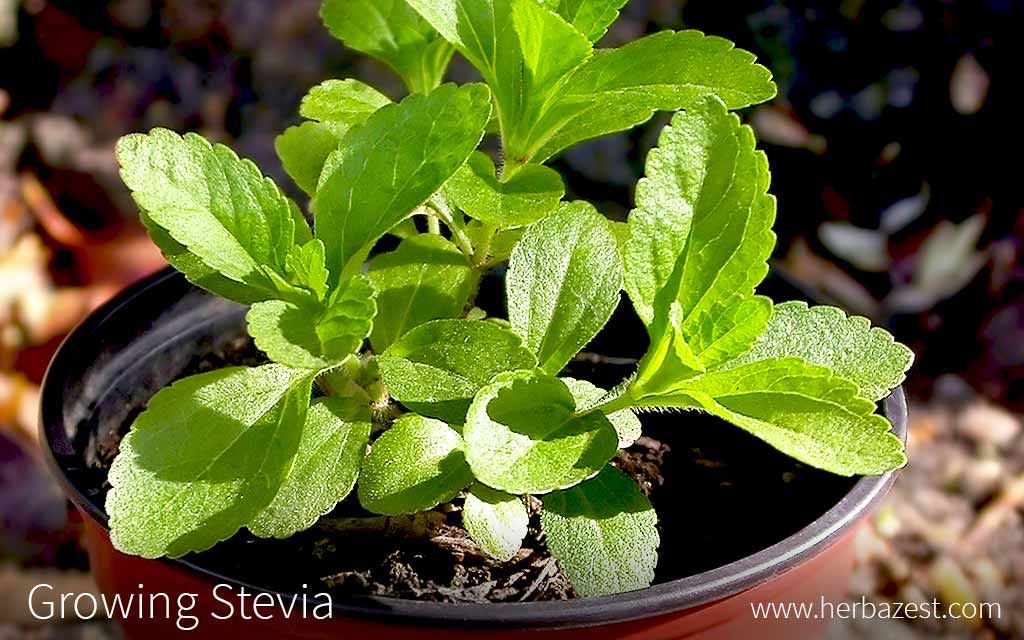This is a detailed close-up image, possibly a poster, featuring a small stevia plant. The plant, bright green with numerous oval, jagged-edged leaves, is positioned centrally, growing in a small, dark red or brown plastic pot partially lined with black. The pot's top edge is visible. The background is artistically blurred, suggesting an outdoor setting due to the natural light illuminating the plant, though no specific background details are visible. The foreground suggests a natural environment with leaves and mulch visible around the plant. Text on the image includes "Growing Stevia" in white letters at the bottom left and "www.herbazest.com" at the bottom right. The colors seen in the image include shades of green, brown, orange, tan, yellow, black, and white.